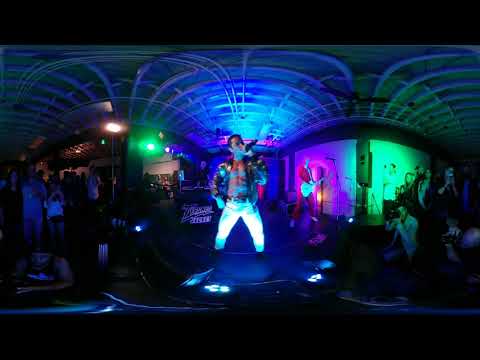In the photograph, a male performer is captured on stage, likely during a nighttime concert or in a dimly lit nightclub. The stage is bathed in an array of colorful lights—green, blue, and pink—that sharply contrast against the dark surroundings. The singer, positioned at the center of the stage, is distinguished by his outfit comprising white pants, an open dark jacket, and no shirt, revealing his chest and abs. He holds a microphone close to his mouth, seemingly in the midst of delivering a performance. To his right, a guitarist dressed in a long red-sleeved shirt and red pants plays an electric guitar, illuminated by a pink spotlight. The audience, scattered to both the left and right of the stage, captures the moment with their cell phones and cameras, their faces lit by the vibrant stage lights.